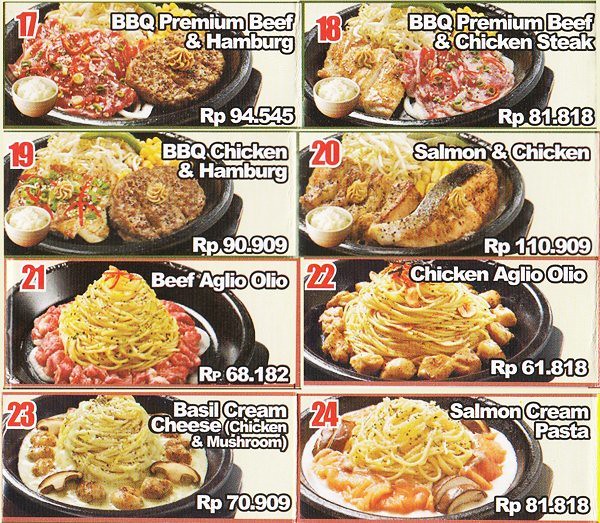The image showcases a detailed photo menu divided into eight sections, each with a numbered and named food item featuring a vibrant picture of the dish on a black plate, accompanied by its price. The menu is organized into two vertical columns with four rows. Starting from the top left, item 17 is "BBQ Premium Beef and Hamburg" priced at RP 94.545, and on the top right, item 18 is "BBQ Premium Beef and Chicken Steak" priced at RP 81.818. The next row features item 19, "BBQ Chicken and Hamburg" at RP 90.909, to the left, and item 20, "Salmon and Chicken" at RP 110.909, to the right. Moving to the third row, item 21 on the left is "Beef Aglio Olio" priced at RP 68.182, and on the right, item 22 is "Chicken Aglio Olio" at RP 61.818. The bottom row presents item 23, "Basil Cream Cheese Chicken and Mushroom" at RP 70.909 on the left, and item 24, "Salmon Cream Pasta" at RP 81.818 on the right. Each item is clearly labeled with red numbering in the top left corner, and the names and prices are in white letters, making for a colorful and enticing display of the restaurant's offerings.